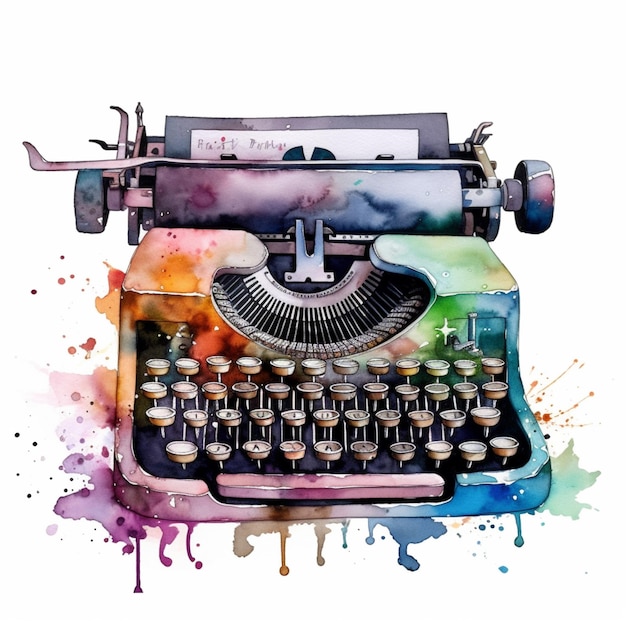This compelling artwork features an old manual typewriter illustrated in a vibrant, watercolor-inspired style. The mechanical typewriter, with its semi-circle of keys and paper roller, stands out against a pristine white background. The entire typewriter is washed in an abstract rainbow of colors, including blues, greens, purples, oranges, and pinks. Cascades of watercolor splatters drip down the sides and bottom, creating a dynamic, almost spray-painted effect with drippy splodges. While a sheet of paper rests in the roller, any text on it remains indiscernible. The juxtaposition of the realistic typewriter form with the chaotic bursts of color bestows a unique sense of beauty and whimsy to the piece. This detailed, colorful artwork melds the familiarity of the old typewriter with an imaginative, abstract presentation, resulting in an intriguingly odd yet aesthetically pleasing image.